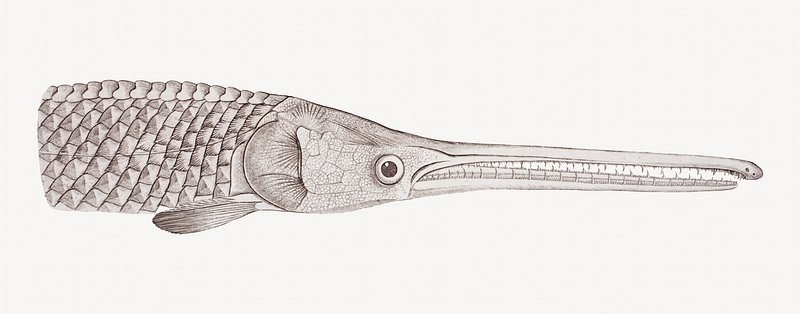This detailed illustration portrays the head of a freshwater fish resembling an alligator gar, a predatory species found in America. The fish's elongated snout is filled with sharp, menacing teeth, invoking a sense of danger that belies its typically scavenging behavior. Its robust, scaly body texture strongly evokes the rugged appearance of an alligator, particularly along its back. The fish's large, eerie eye stands out against the intricate, well-crafted sketch, which showcases delicate, intricate detailing from the gill near the back of its head to the small fins adorning its sides. Only the front half of the fish is depicted, emphasizing its extraordinarily long, tooth-filled snout. The gray background adds depth and contrast, highlighting the fish’s formidable and almost surreal physical adaptations that suggest a complex evolutionary history beyond mere survival.